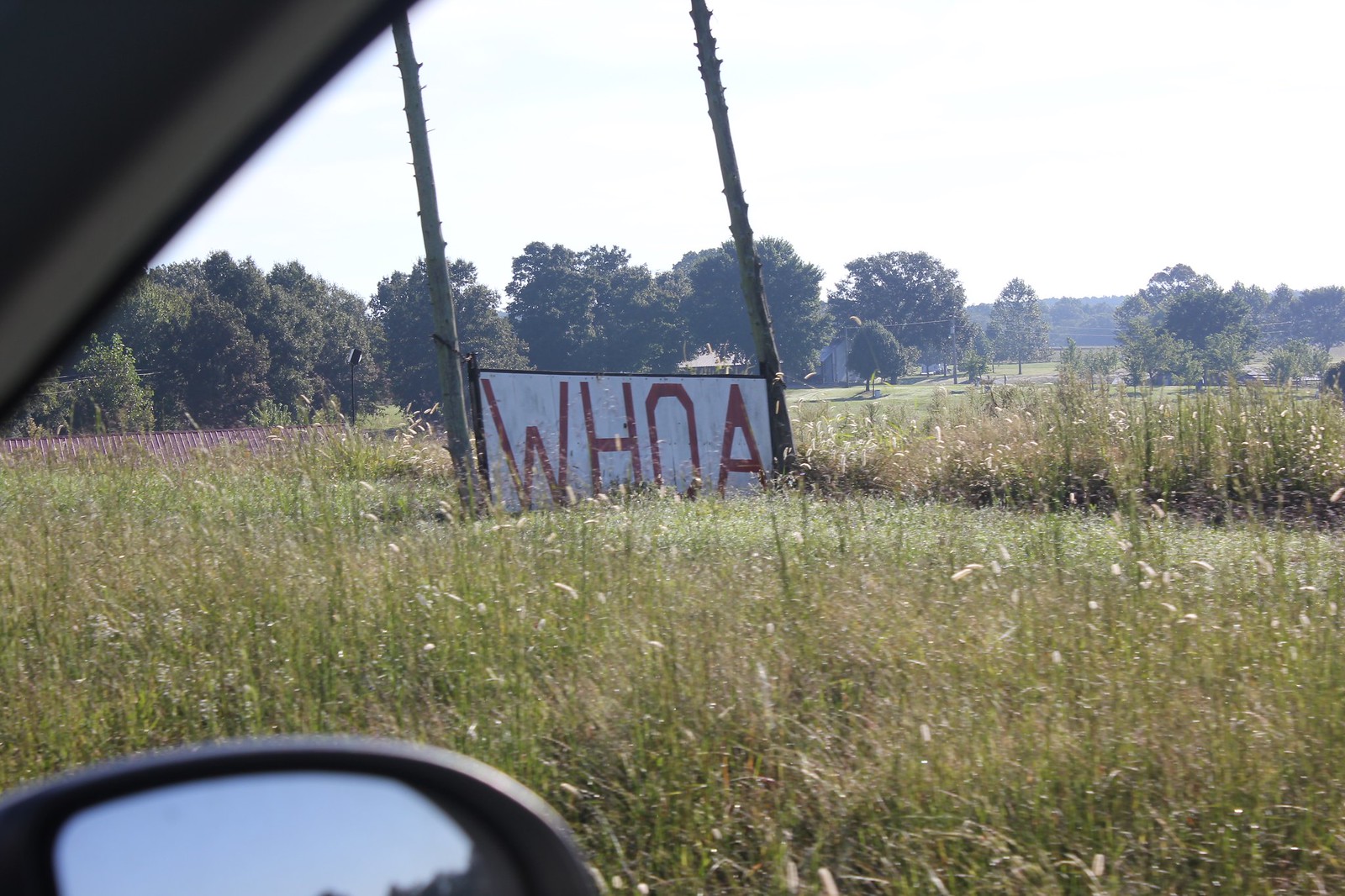Captured from the passenger seat of a car, this outdoor rural scene features a striking, oversized wooden sign displaying the word "WHOA" in bold red letters on a white background. The sign is securely mounted between two tall, slender, and sturdy tree trunks, which have been cut, trimmed, and fixed into the ground. There is an abundance of flat grassland stretching into the distance, accompanied by taller grasses in the foreground. In the far background, large trees and some hills are faintly visible under a loomy, bluish sky. The upper part of the car door and the side mirror appear at the bottom and top left corners of the image, respectively. Additionally, part of a house roof peaks from afar, hinting at human habitation in this tranquil and open landscape.